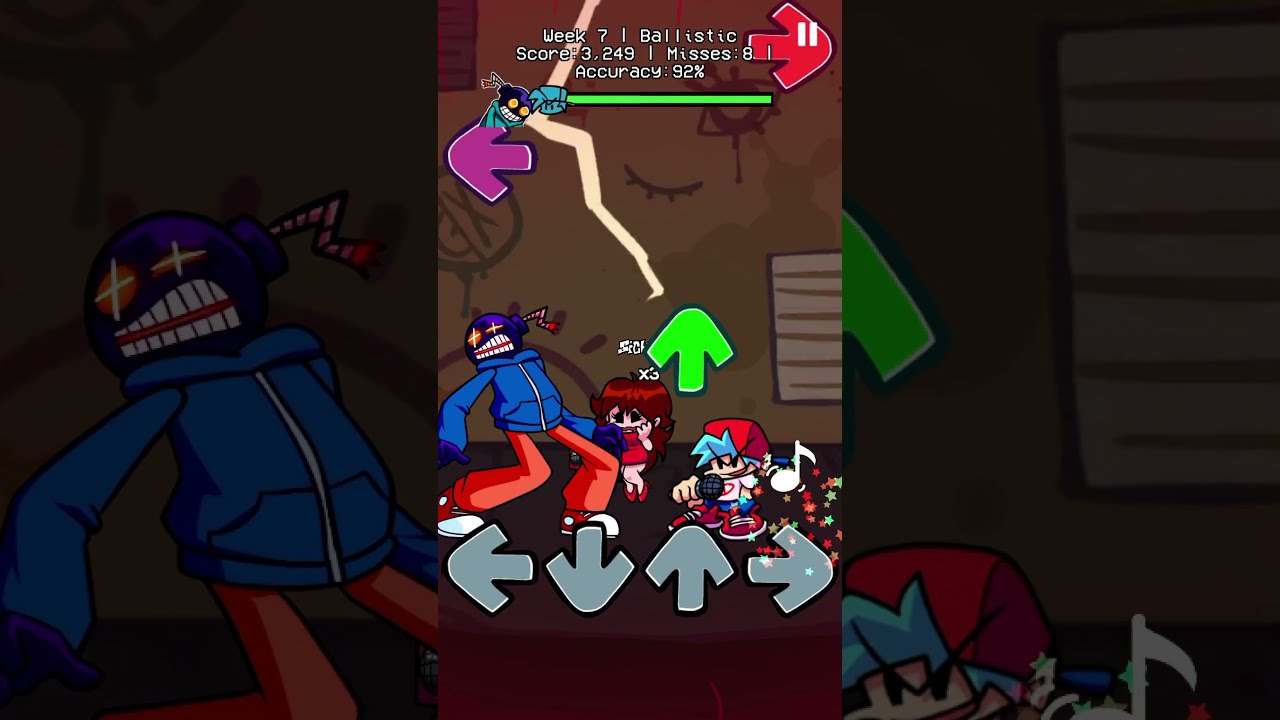The image is a rectangular screenshot from an anime-style rhythm video game, possibly resembling something like Dance Dance Revolution or a music-based game with directional inputs. The central focus of the image shows a smaller version of the gameplay overlaid onto a faded, larger background that is essentially the same scene. 

In the foreground, there are three cartoonish, anime-like characters: a little boy holding a microphone, a large character with a bomb for a head, and a frightened-looking girl with long hair. The background features these same characters but in an enlarged and darkened form, with the boy on the far right and the bomb-headed character on the left. 

At the top of the screen, white text reads "Week 7, Ballistic, Score 3249, Misses 8, Accuracy 92%". There are directional arrows at the bottom of the image indicating possible movements: left, down, up, and right. Additionally, a red arrow pointing to the right with a pause button and a green line under the "accuracy" text are also visible, suggesting game navigation and status indicators. Various arrows serve as clickable or interactive elements for navigating further in the game.